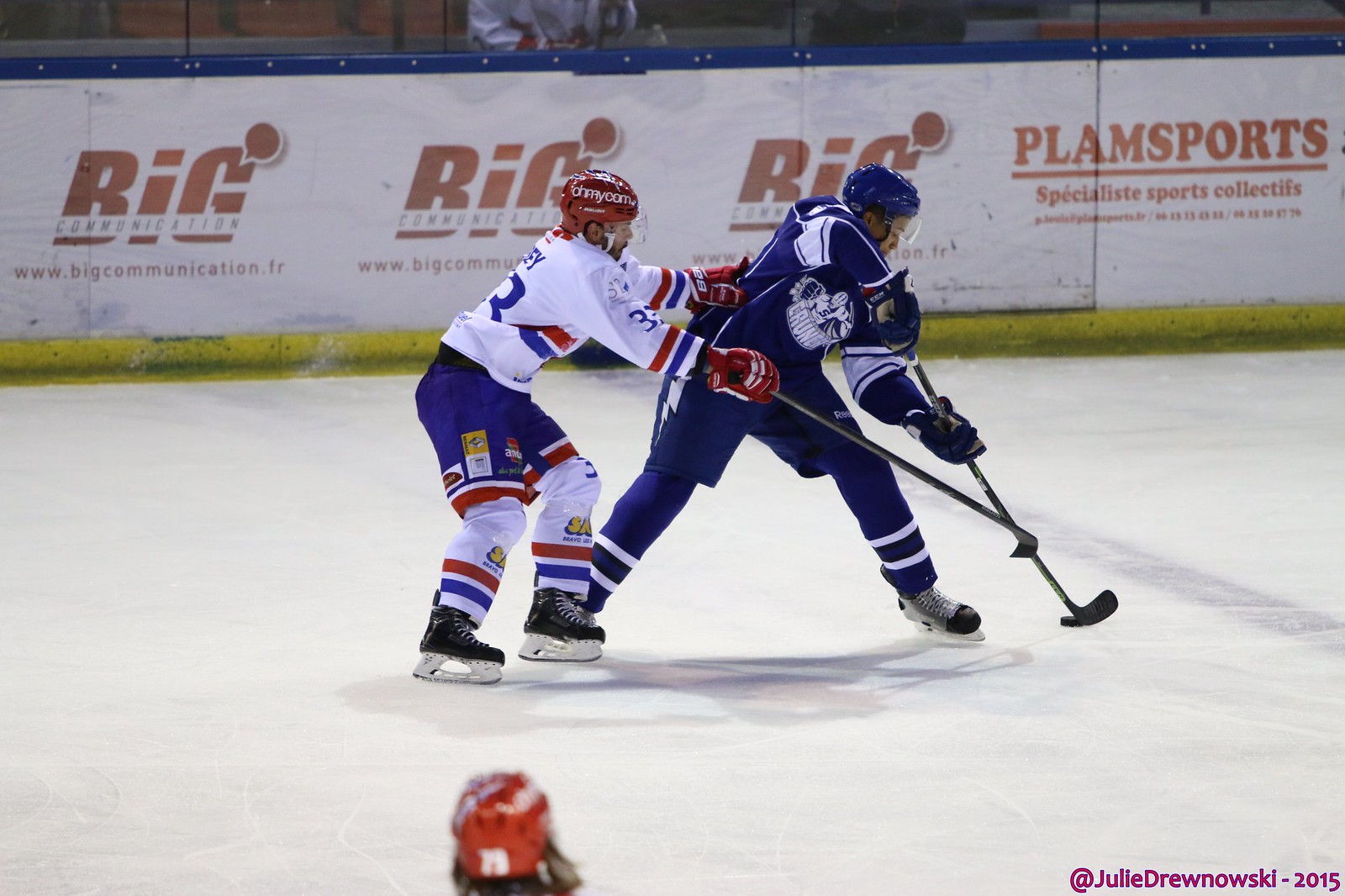This detailed photograph captures an intense moment during an ice hockey game at an indoor rink. At the center of the image, two opposing players vie for control of the puck. On the left, one player is dressed in a white jersey adorned with blue accents, paired with blue shorts. He sports a red helmet and red gloves as he attempts to reach around with his hockey stick to seize the puck from his rival. This rival, positioned to his right, is clad in a blue jersey with white accents, matching blue shorts, gloves, and helmet. Both players are engaged in a fierce contest, their sticks clashing as they battle for dominance.

The ice beneath them is a pristine white, providing a stark contrast to their colorful uniforms. In the background, the boundary wall of the rink is evident, decorated with advertisements. The wall features a white background with a yellow border at the bottom and a blue border at the top. Prominently displayed in red letters is "Big Communication www.bigcommunication.fr," and to the right, "PLAM Sports, Specialist Sports Collectives."

At the bottom right corner of the image, a watermark in purple reads "@Julie Drudnowski-2015," marking the photograph's origin. This vivid scene is a testament to the passion and intensity of ice hockey, frozen in a single, action-packed moment.